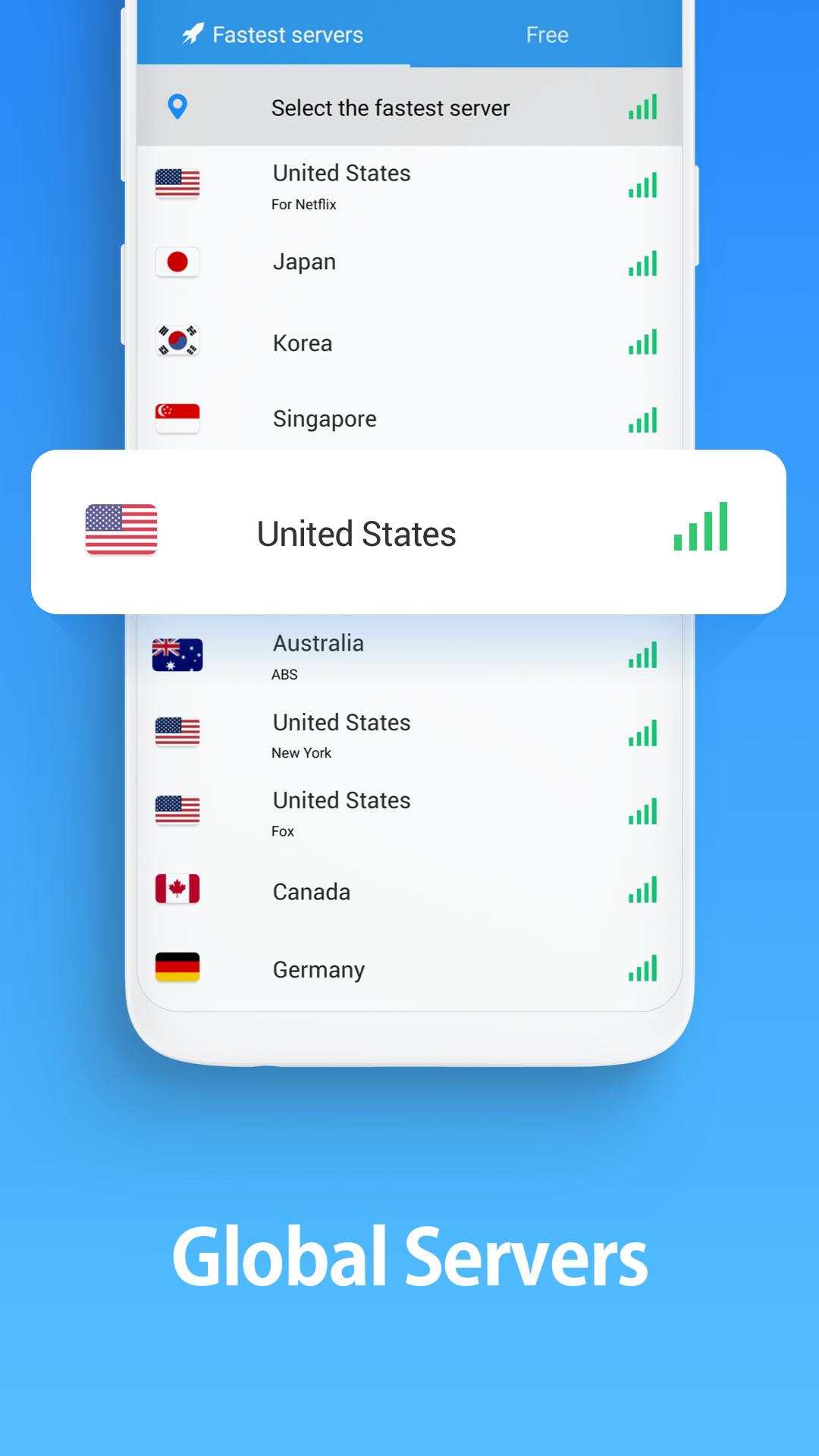A screenshot from an application interface showcasing a selection of global servers. The screen has a blue backdrop and displays various server options with corresponding country flags. At the top of the screen, a banner reads "Faster Servers Free," indicating that users can select the fastest available server. Below the banner, a list of ten servers is visible, including:

1. United States (Netflix) - Flag of the United States
2. Japan - Flag of Japan
3. Japan (again) - Flag of Japan
4. Korea - Flag of South Korea
5. Singapore - Flag of Singapore
6. United States - Flag of the United States
7. Australia - Flag of Australia
8. ABS (United States) - Flag of the United States
9. New York (United States) - Flag of the United States
10. Fox (United States) - Flag of the United States
11. Canada - Flag of Canada
12. Germany - Flag of Germany

At the bottom of the screen, it labels the section "Global Servers." The interface is user-friendly and visually appealing with its organized layout and vibrant colors.